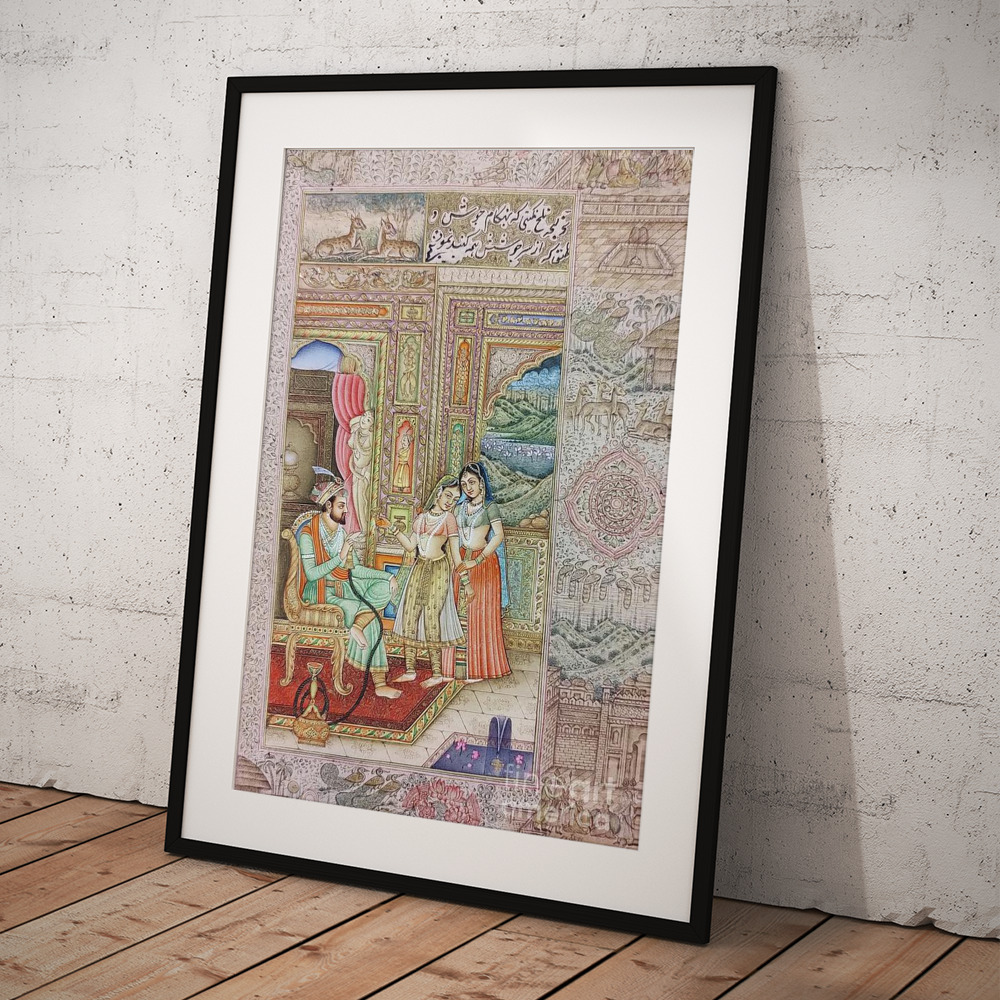The image depicts a framed piece of art displayed against a white, slightly faded cinder block wall, resting on a wooden floor. The artwork is encased in a black frame with a white mat that enhances the illustration inside. The scene within the frame portrays a richly decorated room in a style reminiscent of traditional Indian or Middle Eastern art, featuring muted pastel hues like beige, green, yellow, and red. At the center, a man dressed in elaborate Indian garb, including a grand green outfit and a large, ornate turban, is seated on a throne or chair. He radiates an air of authority, possibly resembling a king, sultan, or pharaoh. Flanking him are two women, adorned in luxurious, traditional attire consisting of crop tops, skirts, veils, and long, intricate jewelry including necklaces and bracelets. They stand on a plush red rug, enhancing the opulence of the scene. The background of the painting is equally detailed, with ornate wall decorations featuring figures like birds, deer, and Arabic inscriptions, adding to the cultural richness of the depicted setting.